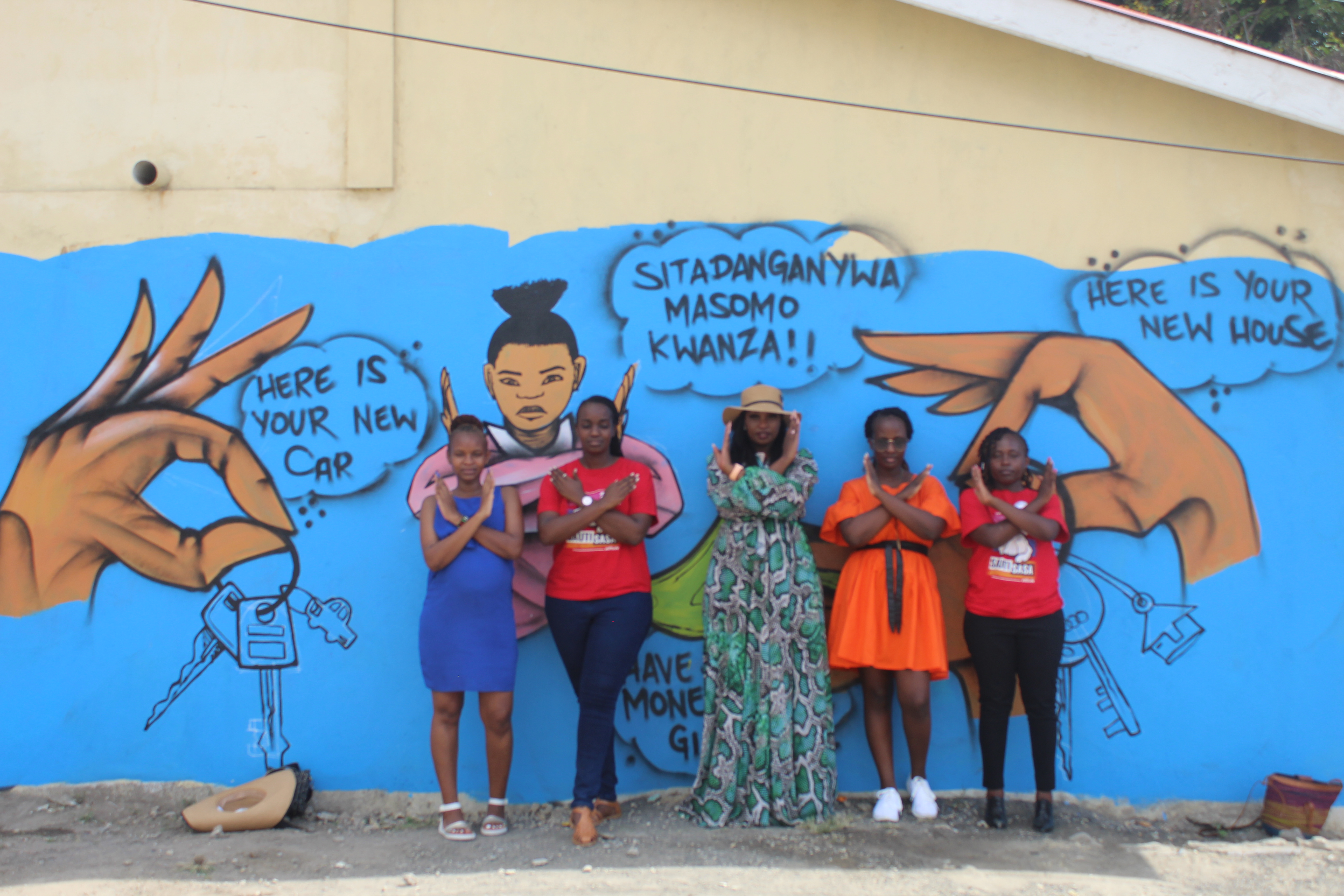The landscape-oriented color photograph showcases five African-American women standing side by side in front of an outdoor mural painted on a building wall. The upper portion of the wall is beige, while a large light blue section stretches horizontally across the bottom. 

From left to right, the women are:
1. A young woman in a blue sleeveless mini dress.
2. A woman wearing a red shirt paired with blue jeans.
3. The central figure, dressed in a long, gray dress with a light green floral pattern, and a hat.
4. A woman in an orange mini dress with a black belt.
5. Lastly, a woman in a red t-shirt and black leggings.

Each woman stands with her arms crossed over her chest in an X formation, mirroring the style depicted in the mural.

The mural itself features two key focal points:
- To the left, a painted black hand holding car keys with a small car charm, accompanied by the text "Here is your new car."
- To the right, another black hand holding house keys with a house charm, next to the text "Here is your new house."

There is additional text above the central figure, which includes the word "Kwanzaa" along with other words in a language that appears to be African, spelling out "Sitadanganywa, Masomo."

The photograph blends the realism of the women and the representational mural art, set against a paved ground with rocks in the foreground.